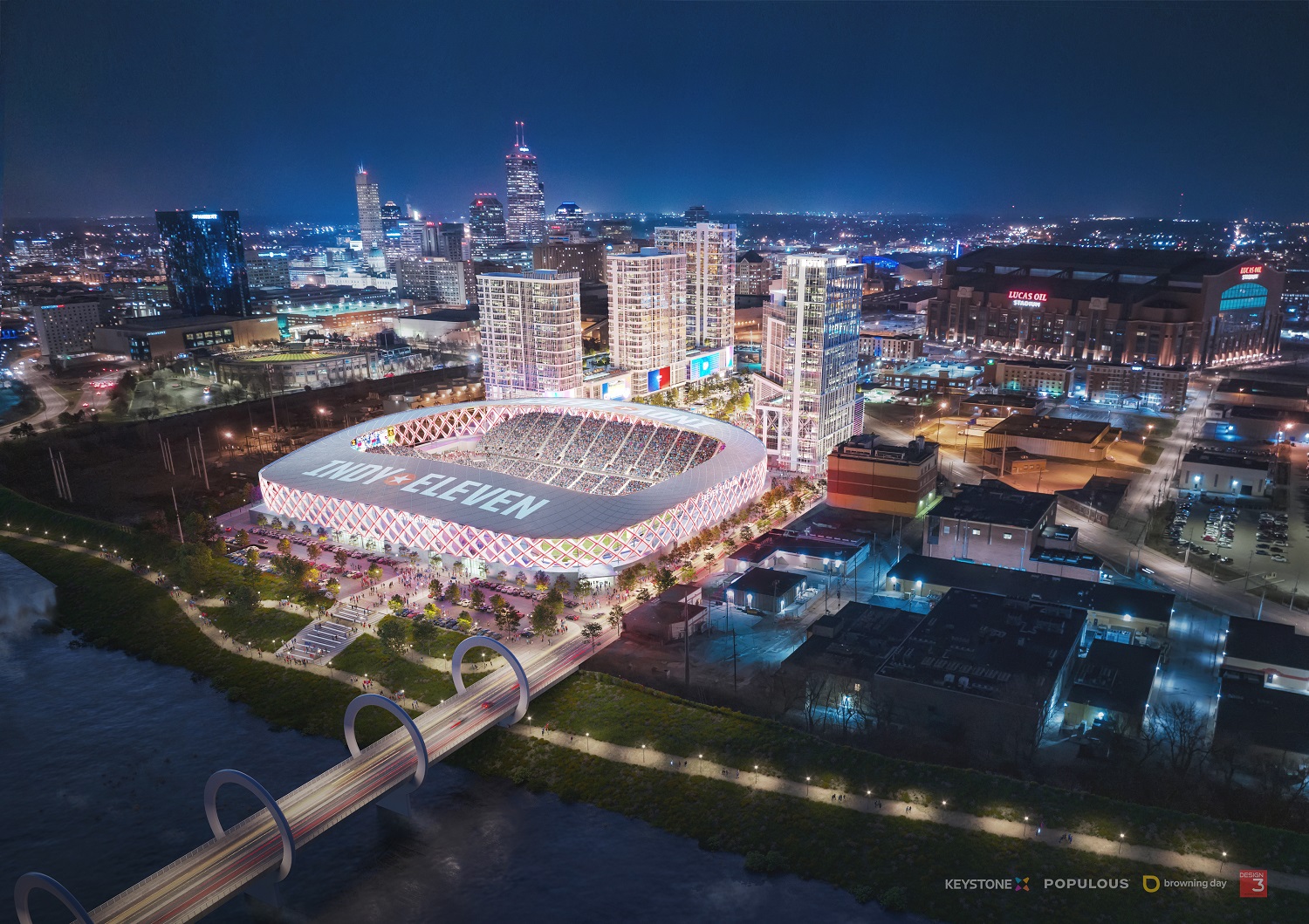This detailed aerial image showcases the illuminated nightscape of a bustling city, presumably Indianapolis. Dominating the center of the photograph is a brightly lit stadium with an open roof, featuring "Indy 11" prominently displayed. The stadium is surrounded by a lattice-like structure and appears to be vibrant and full of life. To the right in the distance, a large brick building is visible, bearing the neon inscription "Lucas Oil Stadium." Further into the horizon, an expansive city skyline looms with towering skyscrapers, all glittering against a night sky turned a deep blue due to the city's radiance. In the foreground, a distinctive bridge characterized by circular designs spans from the lower left towards the stadium, arching over a body of water that hints at a riverbank. Additional details include strings of streetlights connecting various parts of the cityscape, verdant patches of grass fields, and an intricate network of roads and buildings. The image captures the essence of a lively metropolis beautifully lit against the nocturnal backdrop.